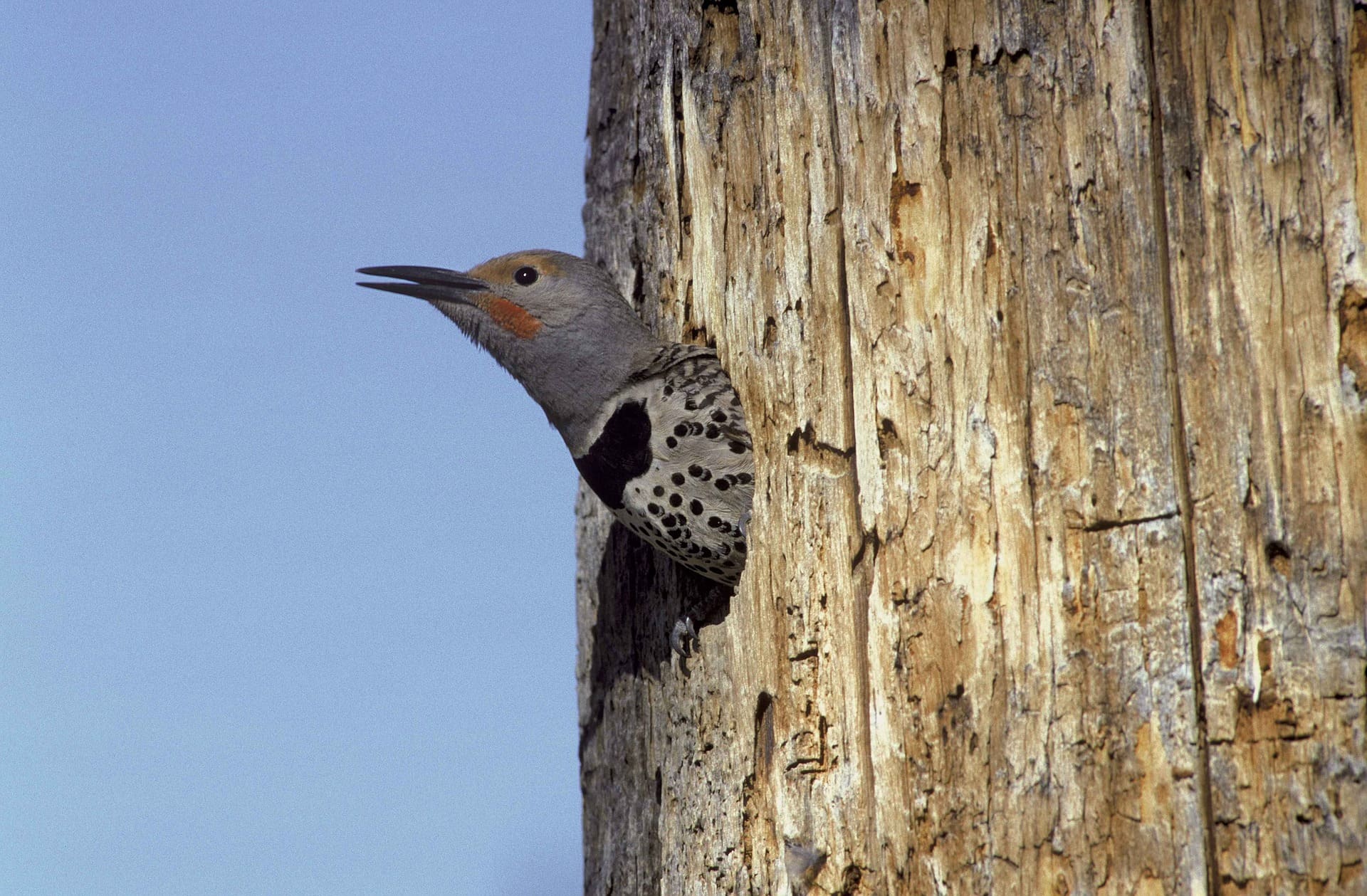A gray bird with distinctive markings is peeking out from a hollowed circle in a tree trunk, which occupies about half of the image. The bird's head is facing upwards, revealing one of its black eyes and a long, sharp beak. Around its eye and beak, there are distinct orange-red feathers. The bird's chest features a black spot resembling a tuxedo bowtie, accompanied by numerous black spots on its body. The surrounding tree bark remains intact except for the hollow from which the bird emerges. The background is a clear, sky blue, adding a serene backdrop to the scene. Little feet or claws can be faintly seen inside the hole.